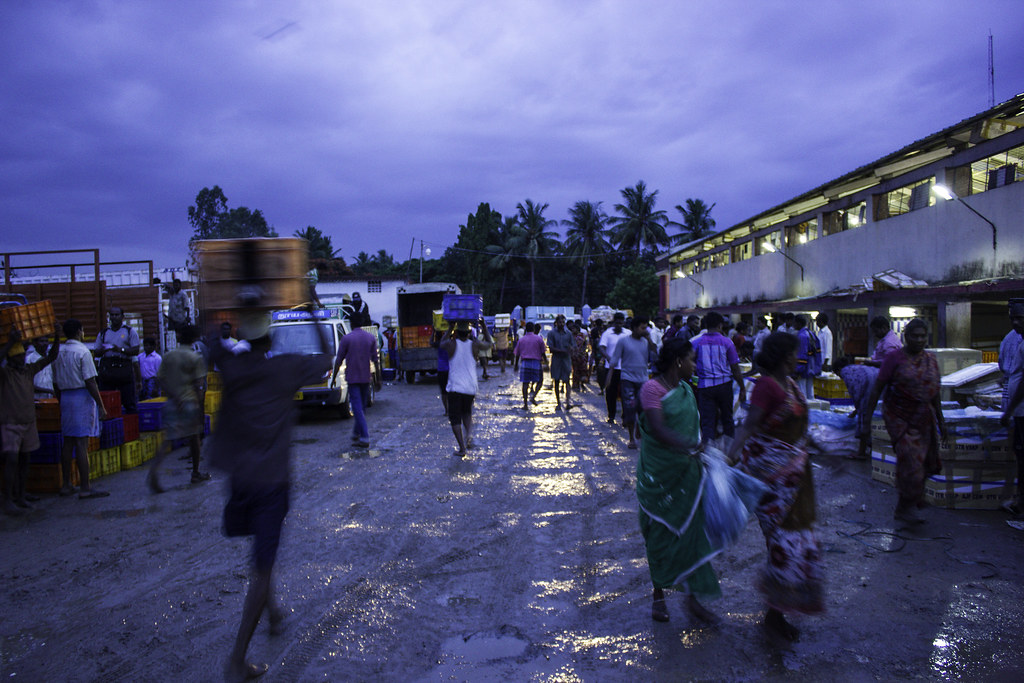The photograph captures an outdoor marketplace during the early evening at sunset in India. The sky is a deepening blue with a few light clouds as the sun has just begun to set, casting a darker theme over the scene. The marketplace is bustling, with around 50 people milling about in various directions on a gravel road. Men and women, many wearing traditional Indian attire and body covers, are engaged in different activities.

On the right-hand side of the image, there is a makeshift, run-down two-story building illuminated by floodlights, casting long shadows across the scene. Women dressed in sarongs and colorful patterned dresses, including one in a green wraparound dress and another in a red and white flowered dress, walk along this building. Men, mostly barefoot and wearing shorts or pants, are seen carrying plastic crates and other items on their heads as they move away from the camera.

On the left-hand side, more men can be seen standing near stacks of boxes, preparing to carry them along the road. In the background, palm trees stretch towards the twilight sky, adding to the serene yet busy atmosphere of the marketplace.